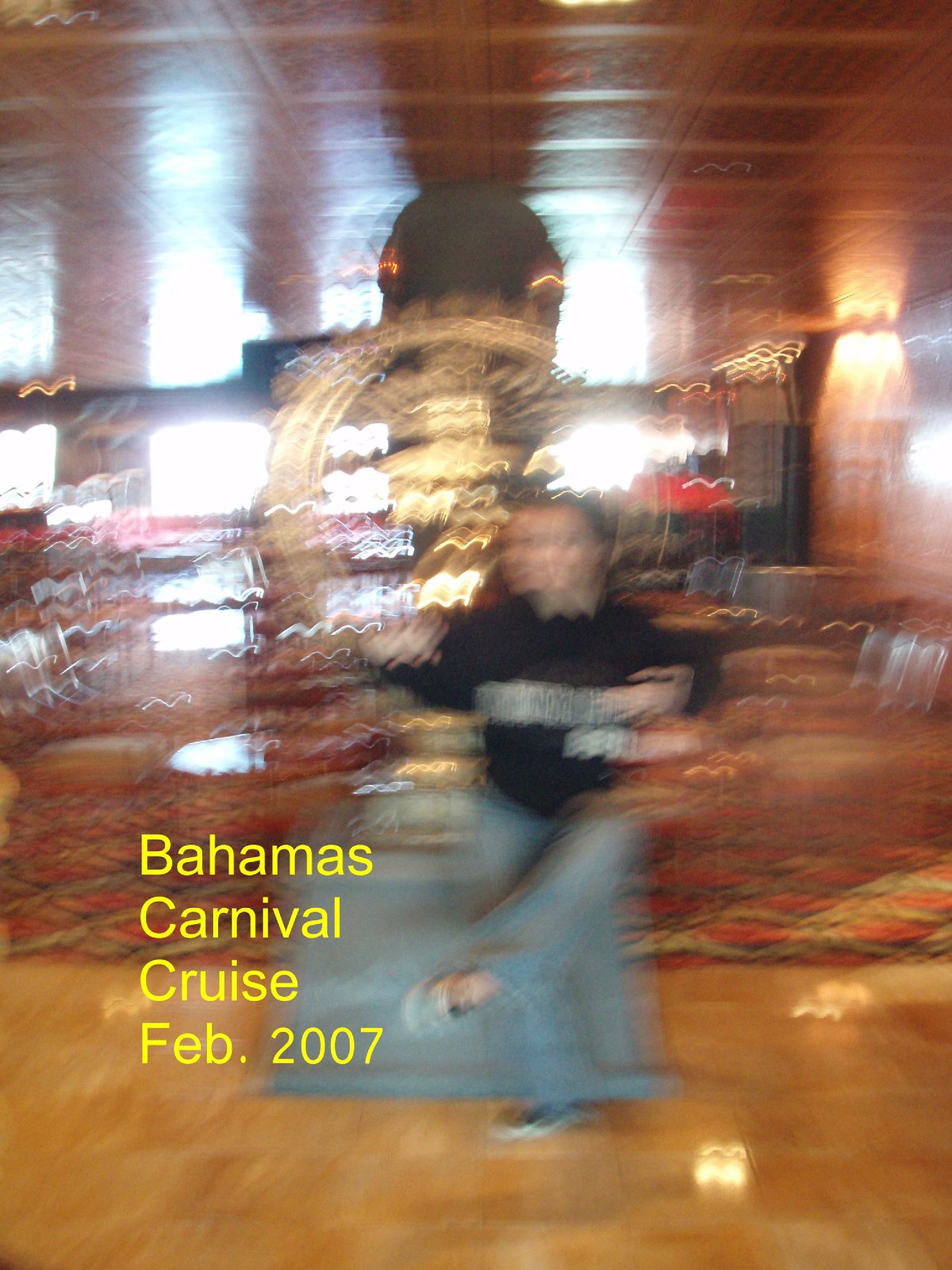This image suffers from extremely low resolution and poor quality, resulting in a blurry, fuzzy appearance. Despite the lack of clarity, there is visible yellow text in the bottom left corner that reads "Bahamas Carnival Cruise Feb 2007." At the center of the image, a person can be discerned sitting on a gray platform. The individual is dressed in a black top and what appears to be gray pants, with shoes that are a blend of black and white. Although the image is quite unclear, the person and their surroundings can still be vaguely perceived.